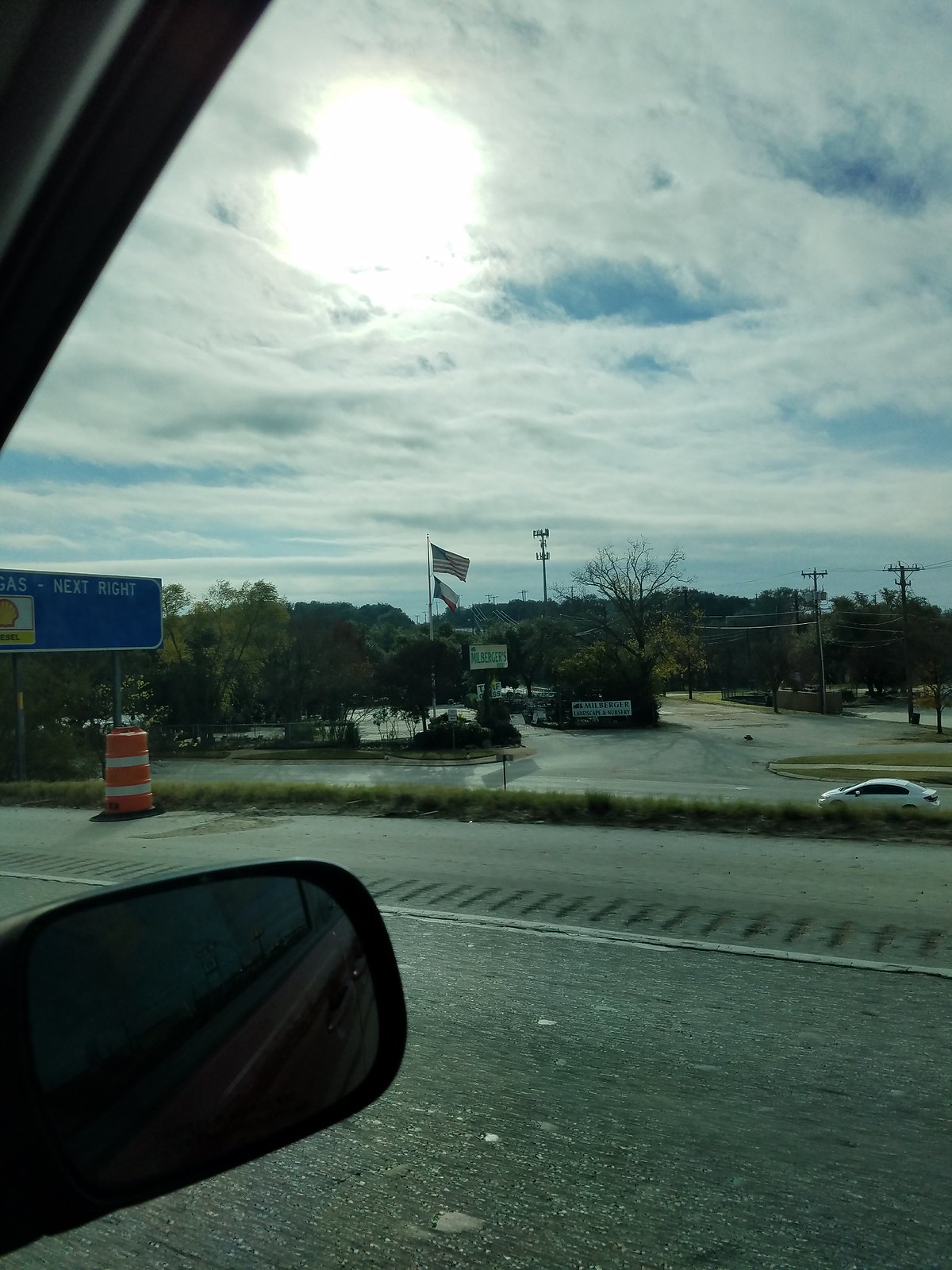The photograph captures a moment from the interior of a vehicle, evident by the inclusion of a rear-view mirror and a segment of the window trim molding in the frame. The perspective is directed outward towards the shoulder of the road. Dominating the roadside is a large, barrel-shaped construction barricade, painted with alternating stripes of vivid orange and reflective white, ensuring high visibility for approaching drivers. Adjacent to the barricade stands a blue road sign, prominently featuring the iconic Shell gas station logo. The sign provides clear and concise directions, indicating that a gas station is located at the next right turn.